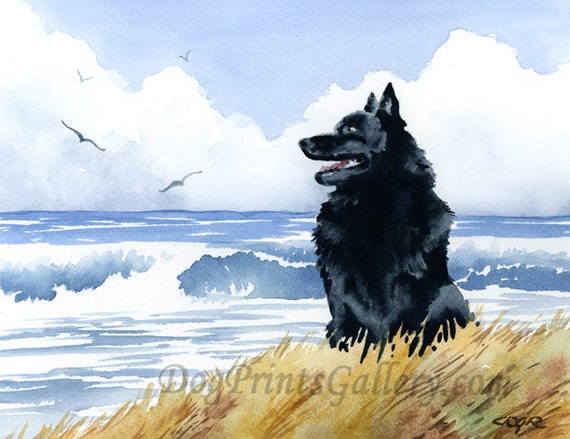In this detailed painting from DogPrintsGallery.com, a solid black dog resembling a shepherd sits on a grassy hill, facing forward with its head turned to the left. The dog's glossy and thick fur shines in the light, and its alert ears suggest an attentive demeanor. Beneath the dog, the grass is depicted in shades of yellowish-brown and green, adding depth to the foreground. In the background, the deep blue ocean, adorned with whitecaps, stretches out towards the horizon. Four seagulls glide gracefully over the water, adding a sense of motion to the serene scene. The sky above is a canvas of thick, fluffy white clouds against a pale grayish-blue backdrop. Barely visible in the grass at the bottom of the painting is the text "DogPrintsGallery.com," along with an artist's signature reading "C-O-G-R."